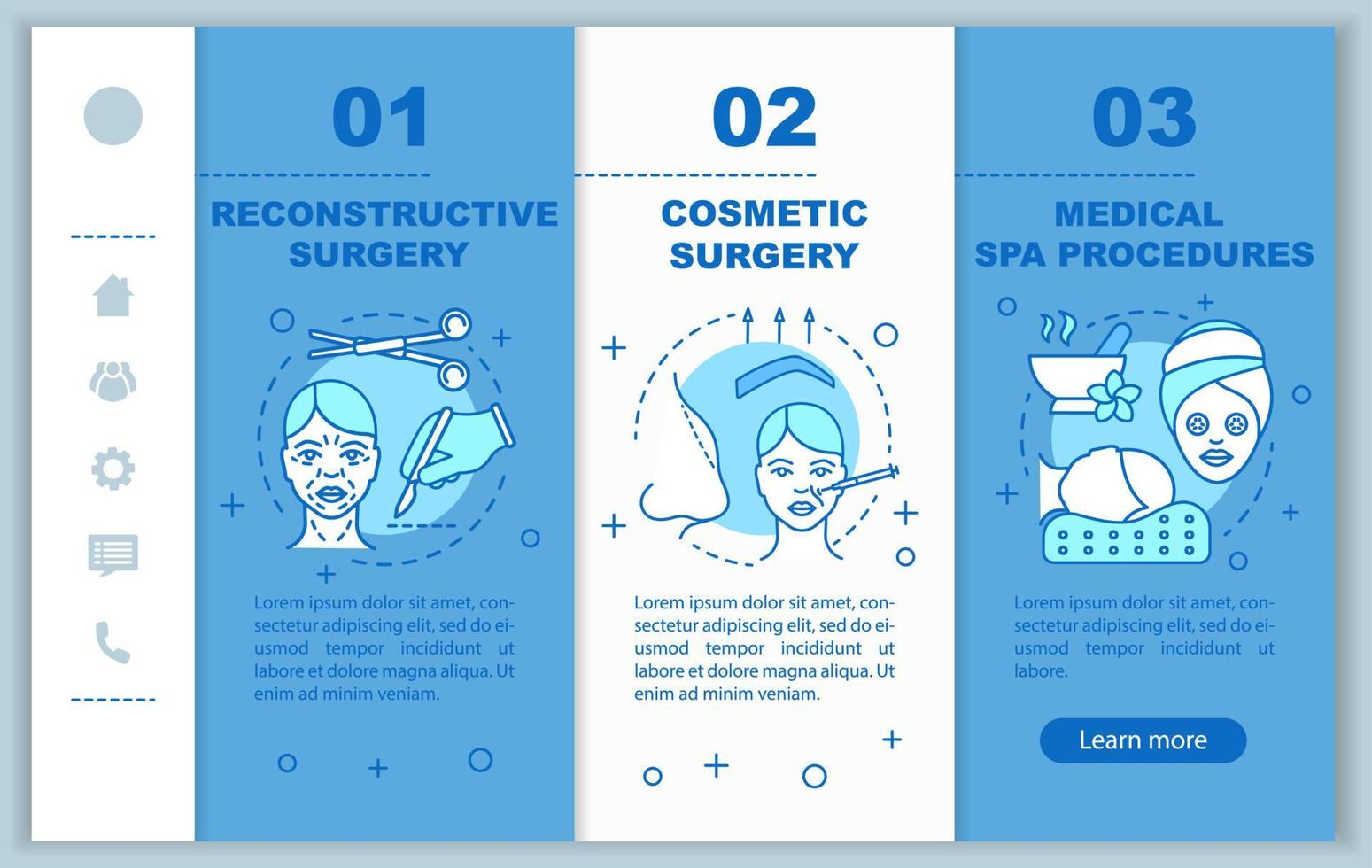The image portrays three distinct medical procedures written in different languages: Reconstructive Surgery, Cosmetic Surgery, and Medical Spa Procedures. In the first section, a person holds a scalpel next to a face dotted with marks, indicating areas for surgical incisions. The second section shows a face encircled and being injected with a needle, while arrows point upwards, suggesting enhancement or alteration. In the third section, there are vivid illustrations: a head with ice cream on top, a steaming mortar and pestle adorned with a flower petal, a head resting on a pillow, and eyes covered with coins, symbolizing death. The bottom right corner of the image features the text "Learn More."